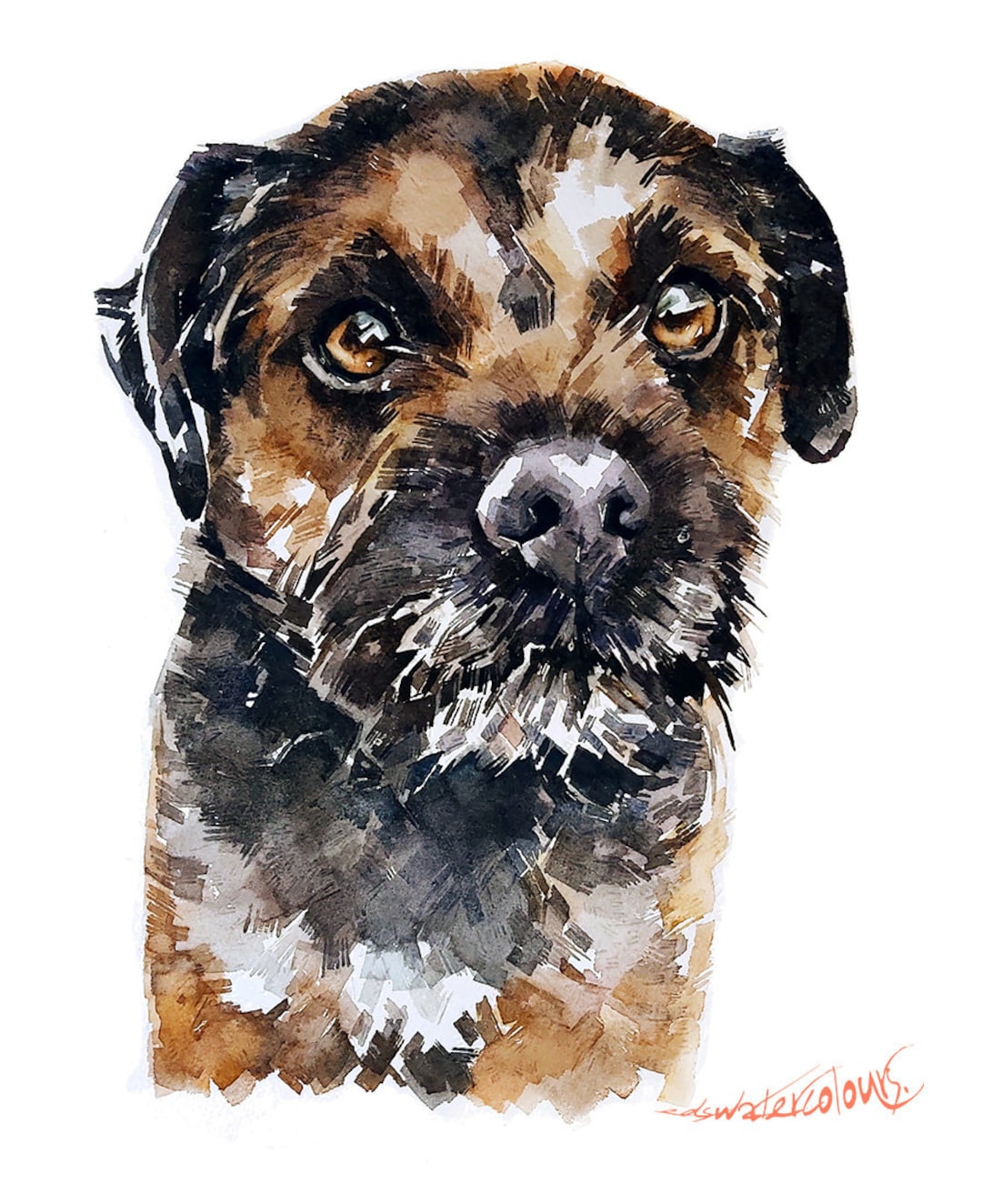This captivating artwork is a watercolor painting of a small, griffin-like dog rendered in a slightly abstract style. The piece features broad, chunky brushstrokes created with a flat brush, which give the dog's fur a distinctive, textured look. The artist has skillfully employed a tricolor palette of black, brown, and tan, with the white background adding a crisp contrast. The dog, facing forward and looking directly at the viewer, has large, expressive caramel-brown eyes with white reflections that add depth and life. The black muzzle, accentuated with highlights, extends to the nose which also glistens with a refined shine. The dog's ears and the top of the head are black, gradually transitioning to brown, while the neck transitions from black to white, then to tan. The chest features a distinctive flash of lighter fur, complementing the overall tan body. The painting is signed in a cursive, brush-like reddish script at the bottom right corner, reading "watercolors," suggesting both the medium and the professional touch of the artist.